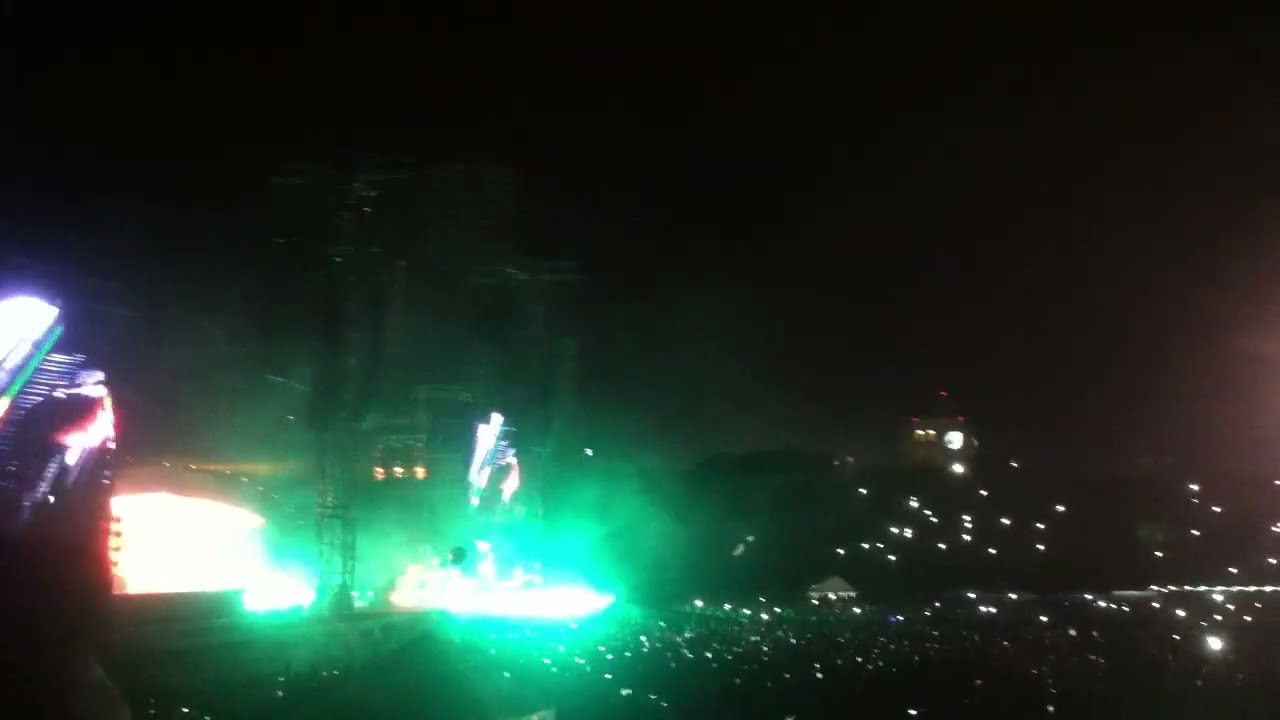The image depicts a large outdoor concert taking place at night in a suburban to urban setting. The overall scene is dark and somewhat blurry, making it challenging to discern specific details. The focal point is a well-lit stage obscured by bright, fiery lights and smoke, with some blue hues among the illumination. Bright lights from what appear to be cell phones and cameras held by attendees create a constellation of dots across the dark expanse, particularly concentrated towards the bottom and middle sections of the image. In the background, faint silhouettes of buildings are visible on the left side, contrasting with the dark sky on the right, which gets progressively darker towards the top. A vertical tower or an angled triangular structure, possibly part of the stage's roof or support, is seen in the middle of the image. Above the stage, a large display screen showcases the performer. The night sky forms a backdrop, with a hint of light on the horizon, adding to the concert's dramatic and vibrant atmosphere.